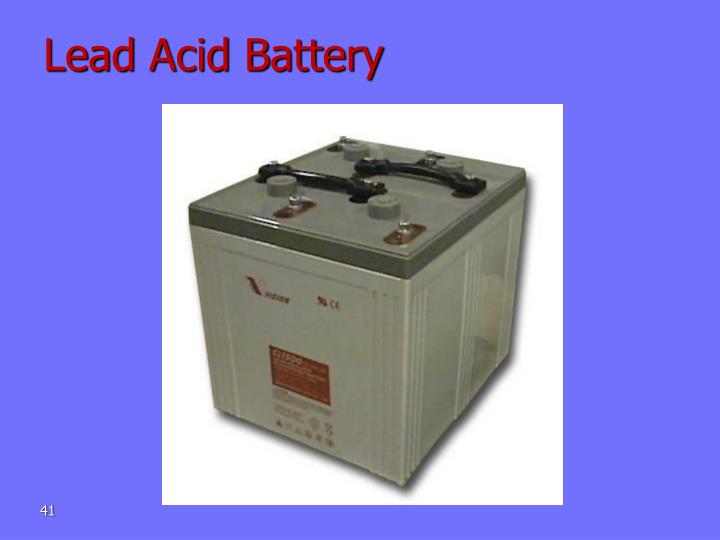This photograph features a lead-acid battery, prominently identified by a red title in the upper left-hand corner that reads "Lead-Acid Battery." The background surrounding the battery is a vibrant purple-violet hue. Situated centrally within the image is a white square frame that houses the lead-acid battery itself. The battery, shaped like a cube, has a two-toned appearance with a light grey body and a dark grey top. On the top of the battery are black handles and several small, shiny silver tube outlets that catch the light. Additionally, a maroon warning or information label is visible on the front side of the battery. The precise positioning of the battery shows it slightly angled towards the right. In the lower left-hand corner of the image, the number "41" is displayed in white text against the purple-violet background, enhancing the overall design of the photograph.